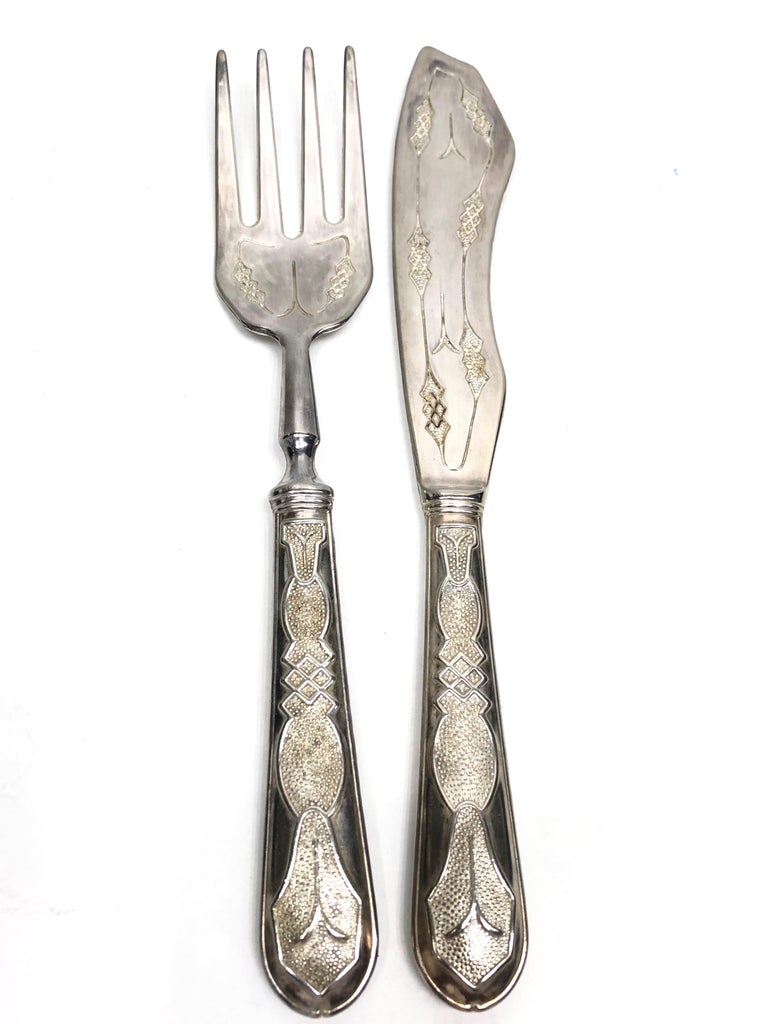The image showcases an elegant and intricately designed silver fork and butter knife set against a pristine white background. The fork is positioned on the middle left, while the knife is situated on the right, both oriented vertically. 

The fork features four pointed tines at the top, adorned with a decorative criss-cross pattern accented with gold designs. The handle transitions into a darker, blackish metal adorned with elaborate engravings, including an oval, diamond shape formed by four squares, and ending with an upside-down leaf shape surrounded by an elongated hexagonal border.

Similarly, the knife’s handle mirrors the ornate design of the fork, with subtle differences in height. The knife blade has a distinctive outlined shape, gently curving outwards in the middle before tapering to a point. Intricate engravings embellish the cutting surface and the handle, which appears to have a black background around the detailed decorations, suggesting the possibility of inset stones or diamonds.

Both pieces of silverware are exquisitely ornate, capturing a sense of timeless elegance and craftsmanship with their enameled designs and gracefully rounded handles.